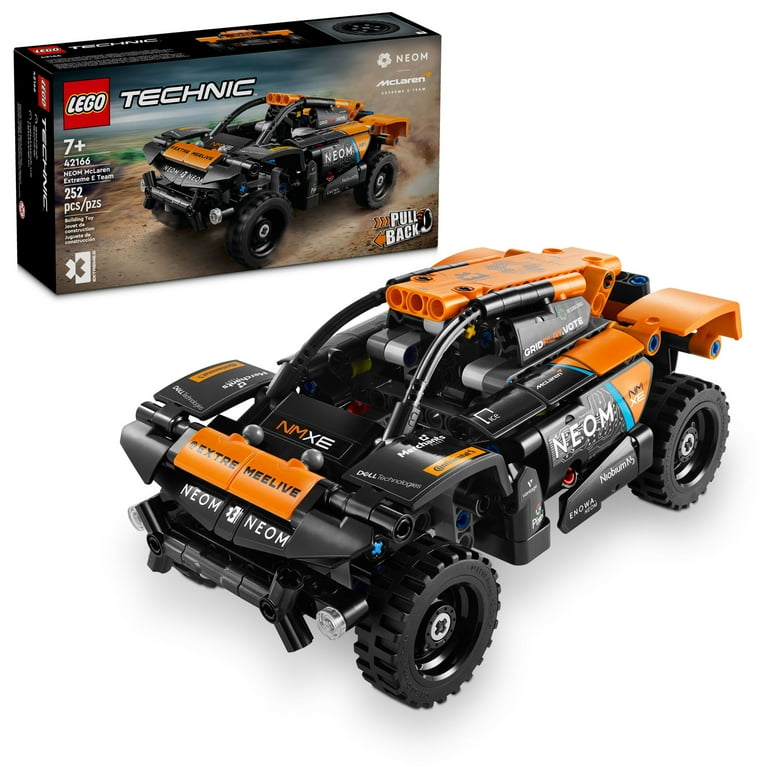The image is a full-color, staged photograph featuring a Lego Technic set against a white background with some shadow. The main focus is a black and orange dune buggy-like vehicle with large, deep-tread off-road tires, distinctively made out of Legos. The vehicle has open windows and orange detailing on the top, front, and back areas. Positioned slightly off-center to the right, the vehicle appears to be oriented towards the left, revealing its two driver's side wheels.

Above the vehicle, slightly to the left, is a photograph of the Lego set's box. In the upper left-hand corner of the box, the iconic red and white Lego logo is prominently displayed, followed by the word "Technic" in white capital letters across the top. The box indicates that the set is suitable for ages 7 and up and contains 252 pieces. In the lower right-hand corner, it mentions a "pull back" feature. Additionally, the box has the branding "Neom McLaren Extreme E-Team" and features an image of the same vehicle, depicted on a dirt terrain.